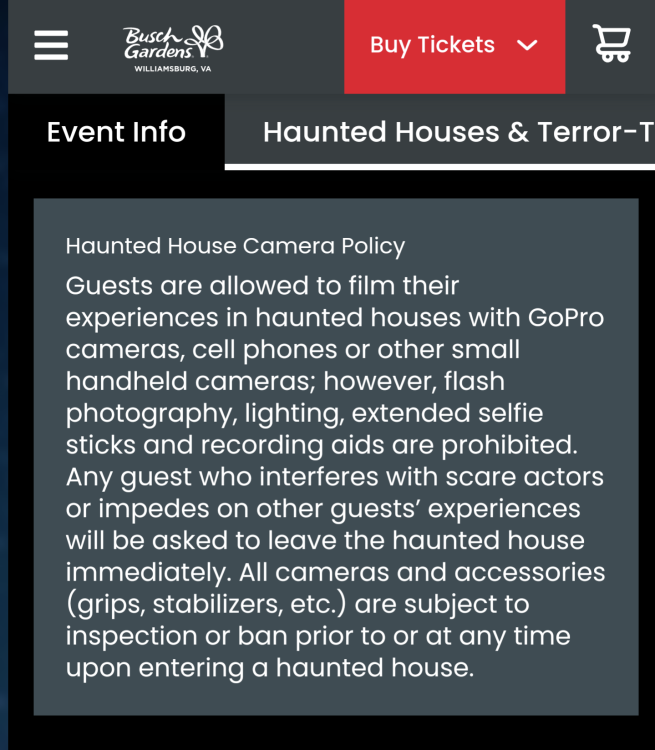The image depicts the Busch Gardens website for Williamsburg, Virginia, characterized by a predominantly gray background. Positioned in the upper right-hand corner is a "Buy Tickets" button, featuring a red background and white font, accompanied by a shopping cart icon alongside it. Navigational elements include a triple-line menu icon located in the top left-hand corner, immediately above the Busch Gardens, Williamsburg, Virginia logo. Two navigational tabs are visible beneath this logo: “Event Info” and “Haunted Houses and Terror,” with the latter currently selected.

The main content area currently displays information regarding the Haunted House Camera Policy. The policy states that guests are permitted to film their experiences within haunted houses using GoPro cameras, cell phones, or other small handheld cameras. However, flash photography, lighting, extended selfie sticks, and various recording aids are strictly prohibited. Guests who disrupt scare actors or interfere with other patrons' experiences will be promptly removed from the haunted house. Additionally, all cameras and accessories, including grips and stabilizers, are subject to inspection or potential bans either prior to or upon entering the haunted house.

This text is presented in white font on a gray square background. The webpage maintains a monochromatic scheme, with shades of gray, black, and white dominating the palette, except for the conspicuous red "Buy Tickets" button. Browsers of the website are likely exploring haunted house options during their visit to Busch Gardens.